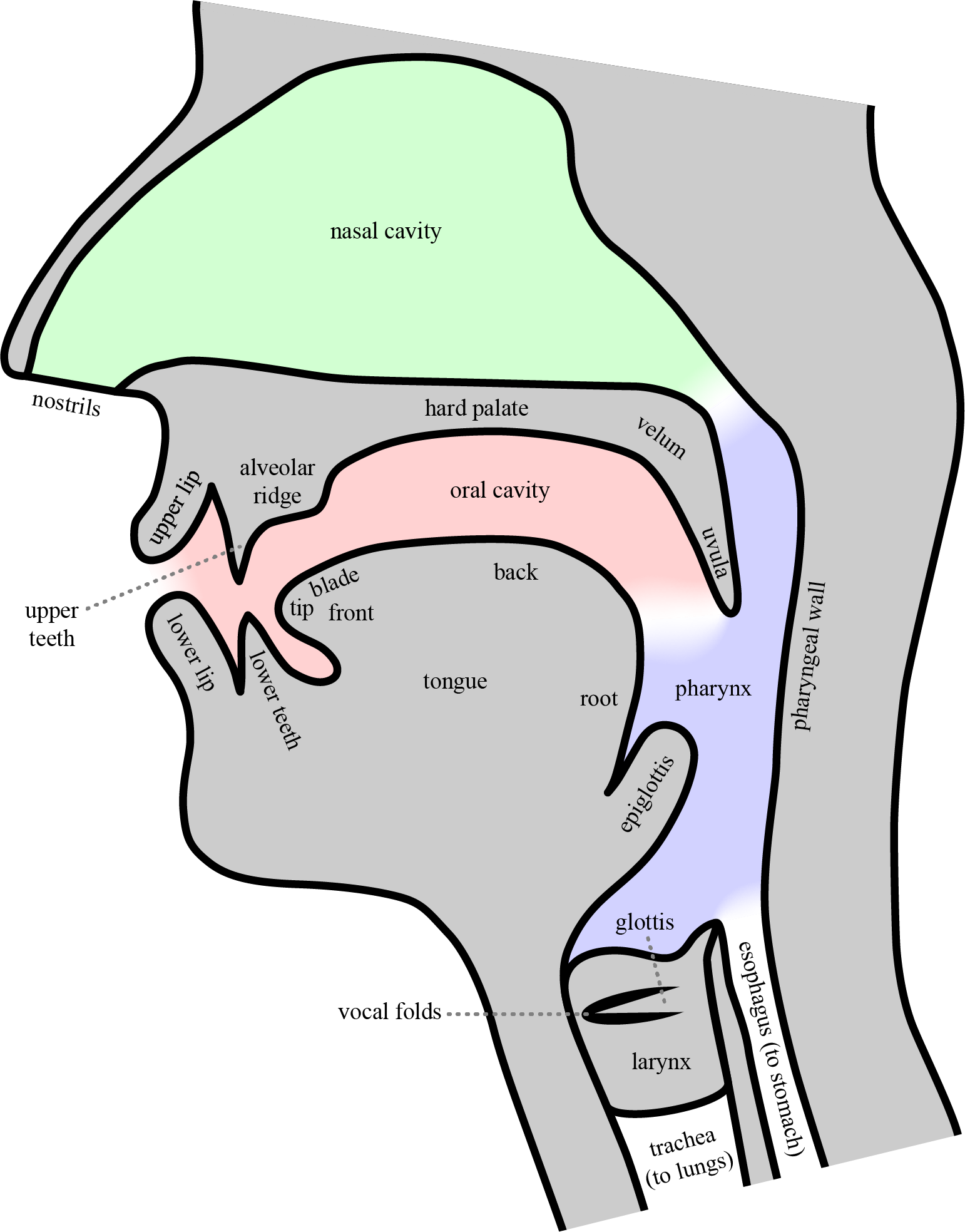This is a detailed and heavily labeled medical diagram of the human head and neck, specifically from the bottom of the eyes to the throat. The digital illustration features a plain white background with a gray-colored depiction of the head and neck, outlined in black. The interior cavities, illustrated in white, highlight the complex anatomy inside the human head and neck. The diagram shows key anatomical structures such as the nostrils, nasal cavity, oral cavity, epiglottis, upper and lower teeth, upper and lower lips, tongue, hard palate, vellum, uvula, pharynx, vocal folds, larynx, glottis, trachea, and esophagus. Some labels are connected with dotted lines, like "upper teeth" and "vocal folds," while others are placed directly on the anatomical features they identify, such as "nasal cavity," "oral cavity," "nostrils," and "tongue." The tongue is further detailed into sections: tip, blade, front, back, and root. The illustration, characterized by its thick black lines and contrasting gray and white color scheme, serves an educational purpose by clearly displaying these features for study and reference.